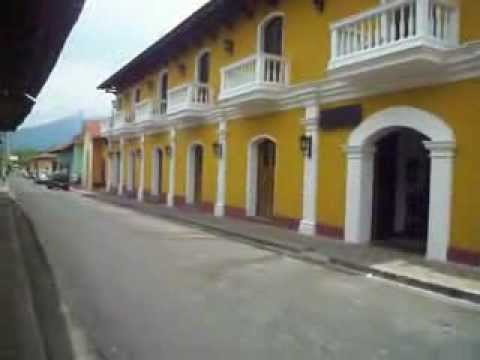The photograph captures a street view dominated by a light gray asphalt road without lane markings, positioned on the left side and foreground of the image. Running along the edges are gray concrete sidewalks bordered by curbs. Towards the top left corner of the image, a light blue sky with white clouds is visible, hinting at the distant outline of a gray mountain. The building on the right side is a yellow two-story structure characterized by multiple white archways housing brown wooden doors on the first floor. The top story features matching brown doors set within white frames, each door opening onto a balcony enclosed with white spindled railings. Various lamps are mounted on white pillars in front of the building, contributing to its European architectural style. Positioned diagonally within the frame, the building draws attention alongside a neighborhood street setting, accentuated by a mix of colors including off-white, full white, light blue, dark blue, various shades of gray, and black.